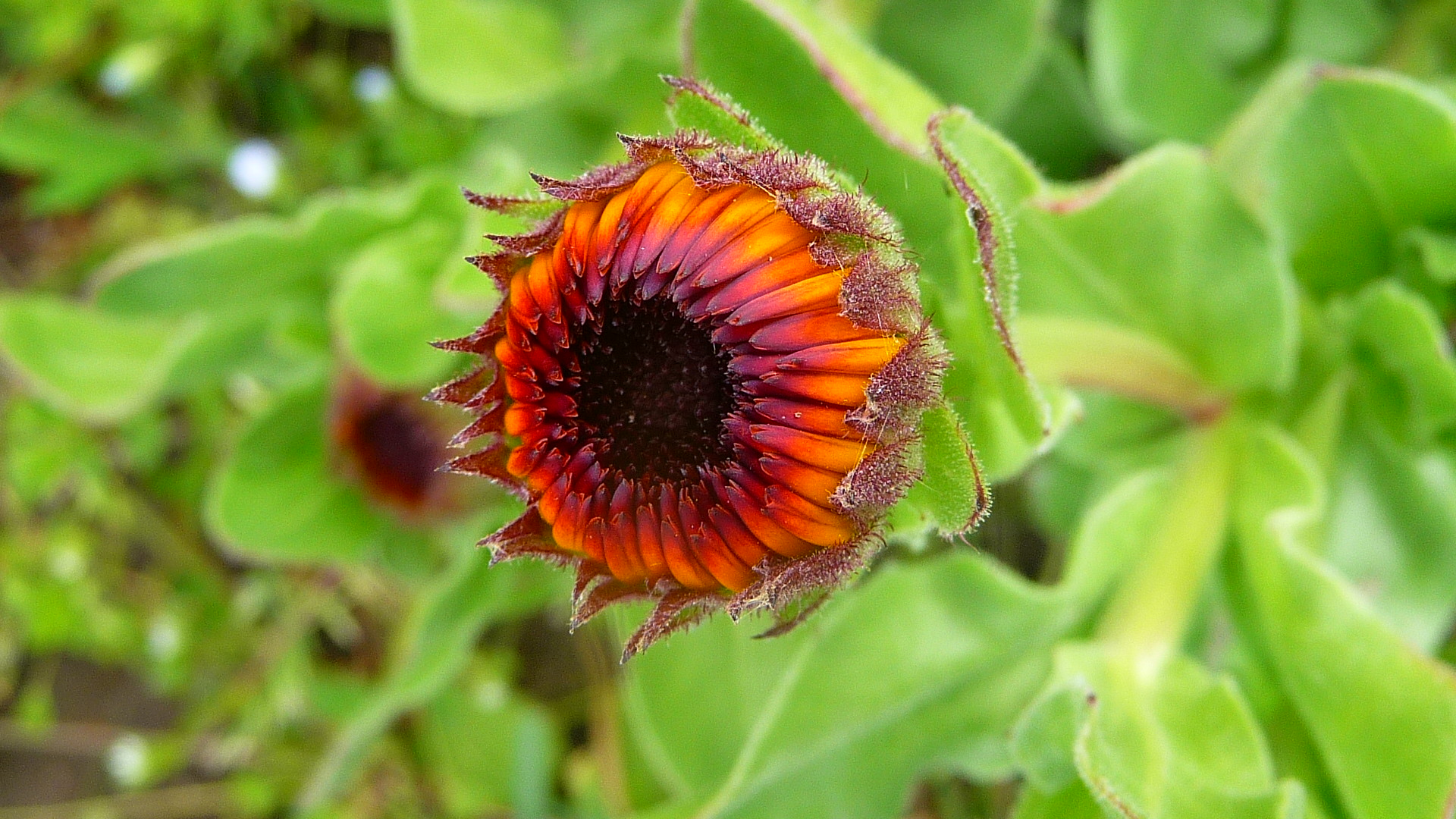This detailed close-up photo captures the vibrant beauty of an unopened flower bud, possibly a black-eyed Susan or coneflower, with striking clarity against a softly blurred green leafy background. The flower sits dead center in the image, with a dark purple center that gradually fades to various shades from deep purple to light purple, transitioning into bright orange, and finally into a yellow hue at the base. The petals are thin and rectangular, radiating outward in a starburst pattern. Surrounding the center are reddish-purple, spiky ridges that appear almost sticky and crystal-like, suggesting they might attract insects. The intricate details, vibrant colors, and the still-condensed petals emphasize the flower’s readiness to bloom, showcasing nature’s splendor up close.